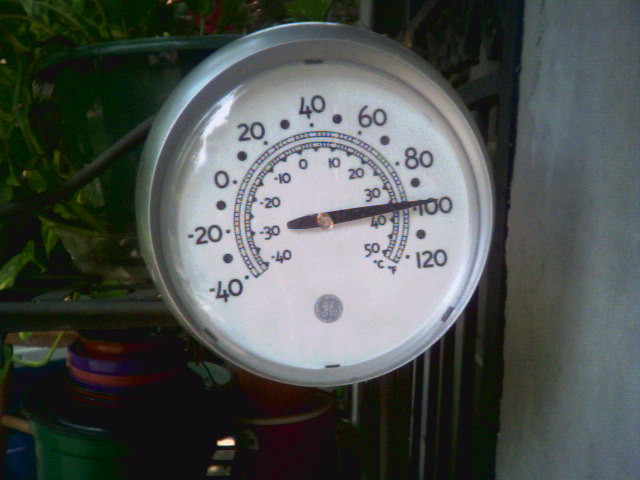A detailed photograph captures a sophisticated ambient scene. Dominating the right side of the image is a blank white wall, providing a neutral backdrop. In the upper left corner, a flourish of green leaves from various plants adds a touch of nature to the photograph. Below this foliage, in the bottom left quadrant, a collection of colorful pots is nestled inside a larger green pot. The vibrant red, blue, and orange pots hold small plants, one of which has begun to sprout.

The centerpiece of the image is a prominently mounted thermometer, affixed to an iron arm extending from the left edge. The iron mounting features three support arms positioned at the top, middle, and bottom for stability. The circular thermometer itself boasts a sleek silver rim. At its core, a white background contrasts sharply with the intricate detailing of the gauge.

At the very bottom of the thermometer, a gray circle is inscribed with the GE logo. The temperature dial is remarkable in its detail: the inner semicircle, open at the bottom, is marked with Celsius measurements, ranging from -40 to 50 degrees, incrementing by 10 degrees. The outer ring provides the Fahrenheit scale, displayed in larger increments from -40 to 120 degrees. The thermometer's needle currently points to 100 degrees Fahrenheit, indicating a notably warm environment.